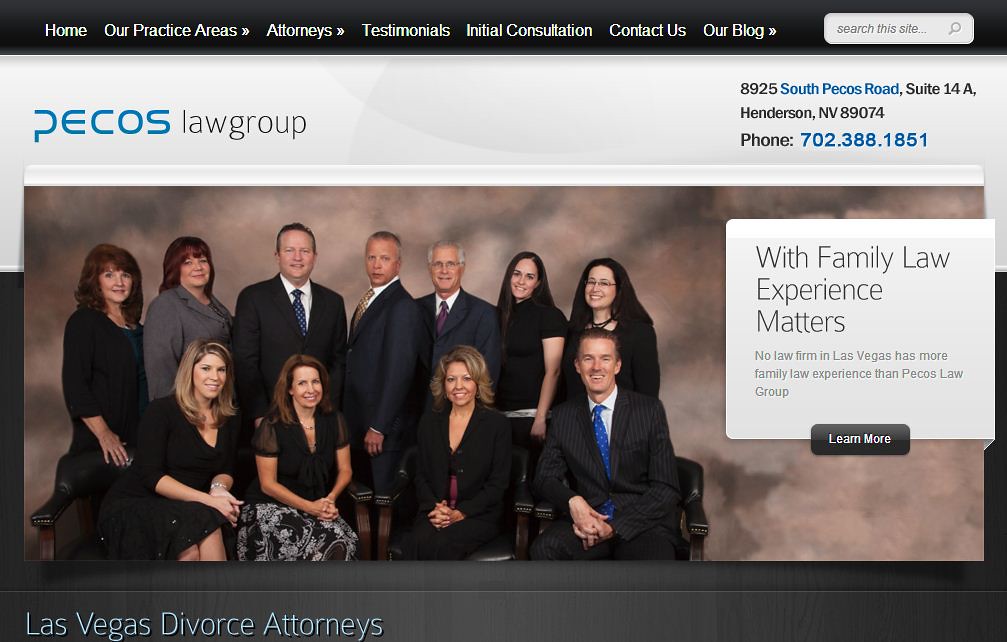This detailed promotional image for PECOS Law Group, taken from a screenshot of their law firm's website, centers on a group of 11 attorneys—seven women and four men—all dressed in business attire of black and gray tones, directly posing for the camera. The background is predominantly black, white, gray, blue, and tan. Surrounding the group, the image displays several text elements: 

- At the top, navigation buttons read "Home," "Our Practice Areas," "Attorneys," "Testimonials," "Initial Consultation," "Contact Us," and "Our Blog."
- On the right-hand side, a promotional blurb reads, "With family law, experience matters. No law firm in Las Vegas has more family law experience than PECOS Law Group."
- At the bottom, it clearly states, "Las Vegas Divorce Attorneys."

The image includes the firm’s address: 8925 South PECOS Road, Suite 14A, Henderson, Nevada, 89074, and their phone number, 702-388-1851. This comprehensive and stylish layout efficiently conveys PECOS Law Group's expertise and available resources.